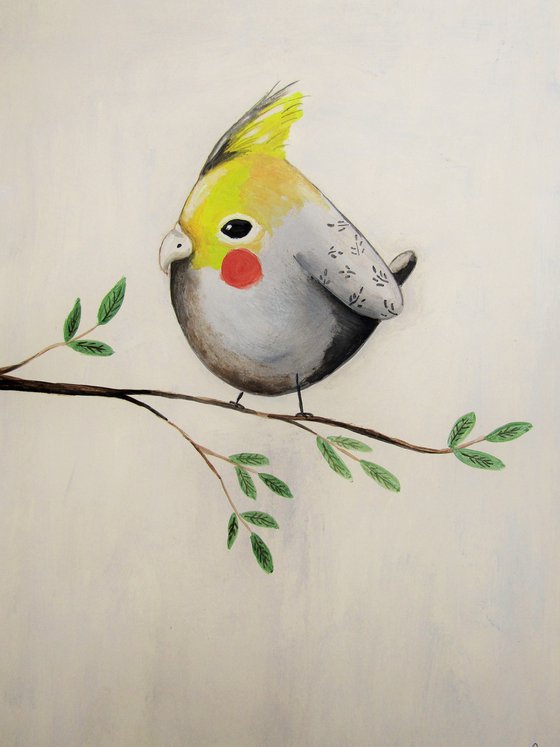This detailed illustration is set against a white paper background that features subtle off-white streaks with hints of orange and gray hues. Extending from the left side of the image is a thin brown branch with lighter brown offshoots. The ends of these offshoots are adorned with clusters of three green, oval-shaped leaves, each exhibiting darker brown veining.

Perched on this branch is a distinctive, somewhat exaggerated bird characterized by its short and stocky build with disproportionately thin stick legs. The bird possesses a striking tall yellow tuft of feathers on its head and features a sideways almond-shaped black eye. Notably, there is a prominent red dot on its cheek, reminiscent of a cockatiel’s markings. The bird's body is white with a slightly darker shading on the underside and speckled patterns along its short gray wing. Its head is yellow, which extends around the eye area, and it has a noticeable red circular mark below one eye. The presence of a single breathing hole in the bird's beak adds a touch of realism. The branch appears to bend slightly downward, presumably under the bird's weight, adding to the dynamic quality of the composition.